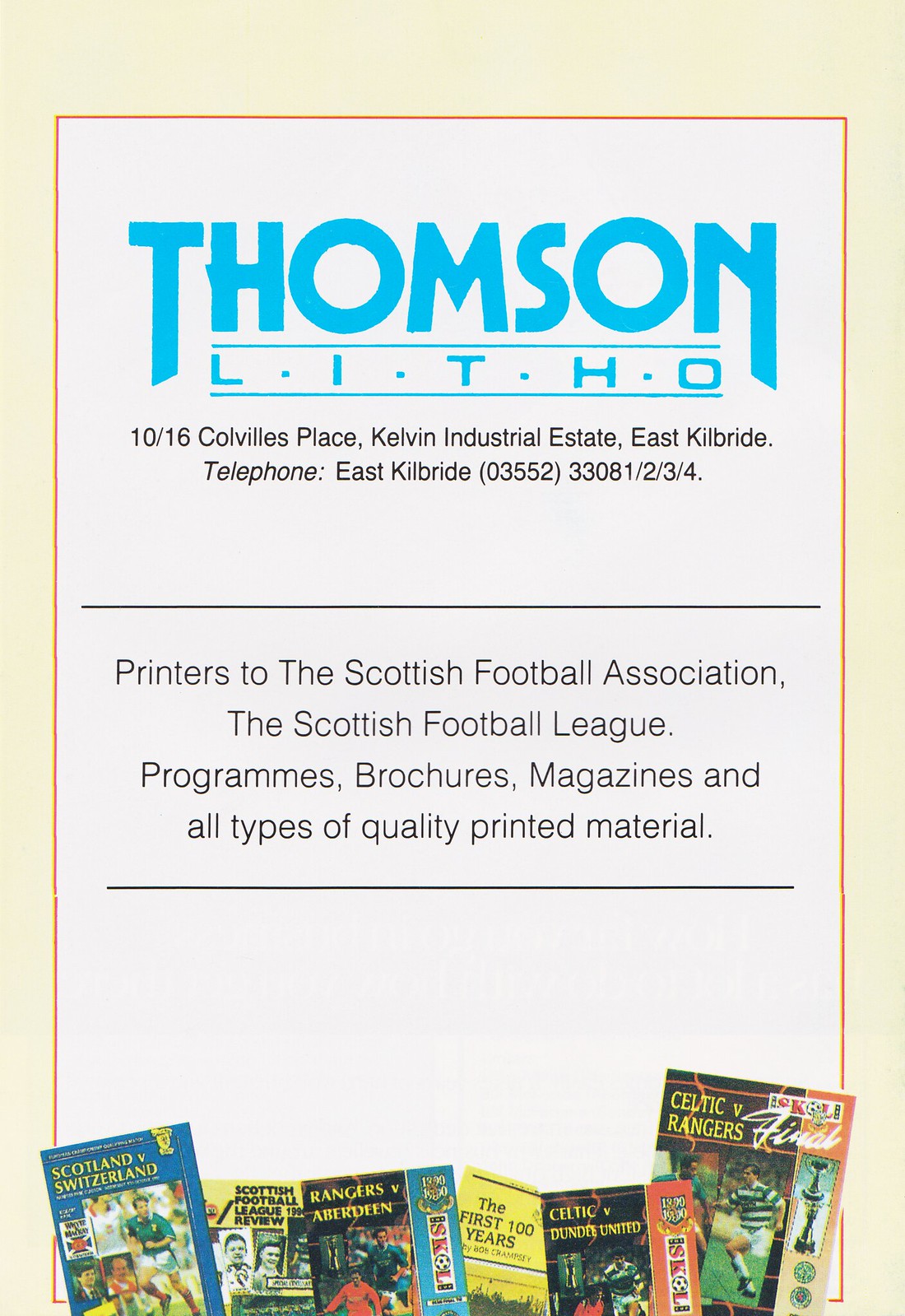The image is an advertisement that features a faded, nostalgic design reminiscent of the 1980s or 1990s. It has a soft yellow outer border, a thin orange inner line, and a white background. At the top, in large, bold blue font, it reads "THOMPSON," followed by two horizontal blue lines framing the word "L-I-T-H-O," with each letter separated by blue dots. Below this, in smaller black font, it lists the address: "10-16 Colville's Place, Kelvin Industrial Estate, East Kilbride," along with the telephone number formatted as "East Kilbride 03552 3308 1/2/3/4." Within two thin horizontal black bars, the text reads, "Printers to the Scottish Football Association, the Scottish Football League, programs, brochures, manuals, and all types of quality printed material." At the bottom of the image, there is an array of old Celtic and soccer magazines, reinforcing the vintage character of the advertisement.